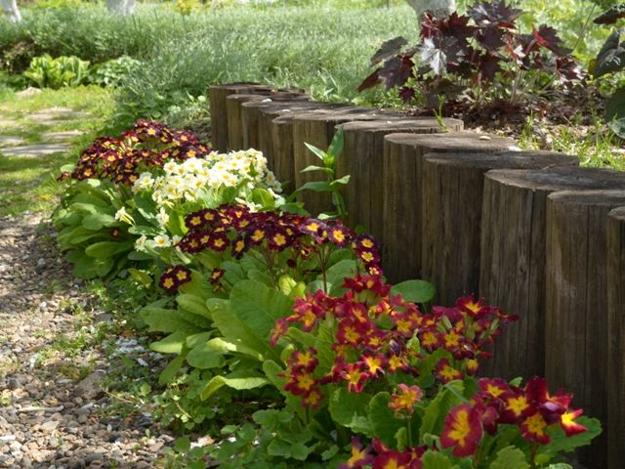This detailed photographic image captures a meticulously cultivated garden area. At the forefront, a row of vibrant flowering plants thrives, each adorned with large green leafy foliage. The flowers, all uniform in size, exhibit a striking array of colors: those with pink outer petals and yellow centers, others bearing maroon outer petals with yellow centers, and some showcasing white petals with yellow centers, with the maroon flowers appearing again at the end of the row. This floral display is planted in front of a distinctive wall constructed from large, untreated tree stumps, each cut to the same size and placed closely side by side. The rustic, natural texture of the stumps contrasts beautifully with the colorful blooms. To the right and extending into the background, a tall oriental maple tree with dark red or purple leaves adds a dramatic accent to the scene. Beyond the main planting area, the photo reveals additional green plants, including hostas and tall, thick grass stretching into the distance. A gravel pathway weaves through the garden, enhancing the serene, cultivated atmosphere.